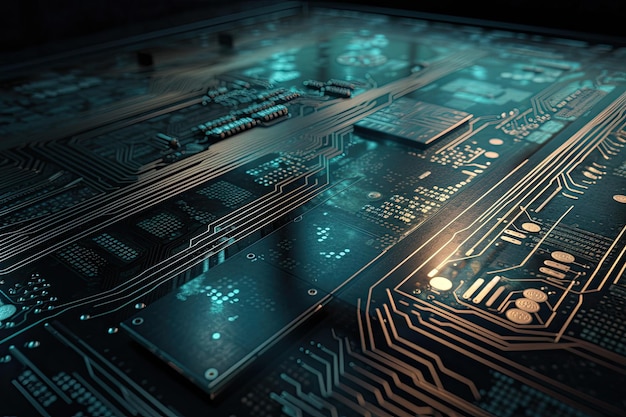This image is a detailed CGI render of a close-up view of a motherboard, specifically a circuit board, with a rectangular shape where the longer sides run horizontally. The board's overall color tone is green with darker, almost black edges, indicating a shaded or dimly lit indoor setting. The circuit board's surface is populated with an array of electronic components, including a central area featuring intricate gold circuit lines arranged in parallel running diagonally from the lower left to the upper right. 

On the center left of the image, there's a noticeable region with small metal rings, designed for other components to screw into and integrate into the circuitry. Also, in this area and a bit above it, a series of transistors can be seen, though they are somewhat out of focus, making detailed observation challenging. Towards the bottom left, there are a few prominent metal endpoints where the circuitry lines terminate, adding to the complex layout of the board.

A square computer chip is prominently situated in the upper left, with smaller plug-in-like rectangular components dispersed around. Additionally, on the center right, there are gold-shaped circles prominently visible. The image seems to capture various reflections, including a subtle yellow light, giving the board a reflective sheen, and an aqua-blue glow emanates from underneath, possibly from embedded LEDs. The flash illumination from the camera also highlights the metal surfaces, contributing to the overall vivid and tech-rich aesthetic of the render.